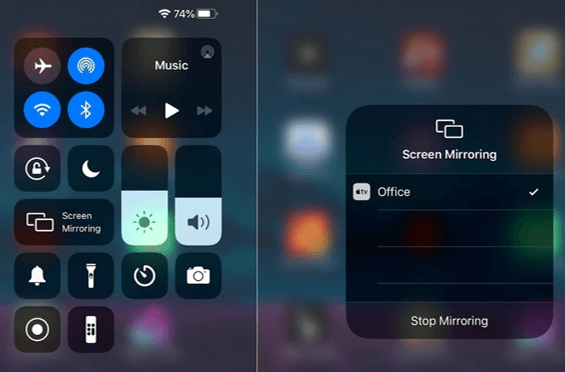The image is a screenshot of the Control Center from an iPad or iPhone, accessible by swiping down from the top-right corner of the device. The left side of the Control Center features various widgets, including icons for Airplane Mode, AirDrop, Wi-Fi, and Bluetooth. Below these, there is a section dedicated to music controls. Further down on the left, there is a brightness adjustment slider, while on the right side, there's a volume adjustment slider. To the left of the volume slider are the screen rotation lock, Do Not Disturb button, and the Screen Mirroring option. Additionally, there are icons for the notification ringer, flashlight, timer, camera, screen recording, and a button for accessing Memoji or other emoji options.

On the right, another section of the Control Center is expanded, showing the Screen Mirroring options. At the top of this section, the "Screen Mirroring" title is displayed, followed by the Apple TV logo with the label "office" and a check mark next to it, indicating an active connection.